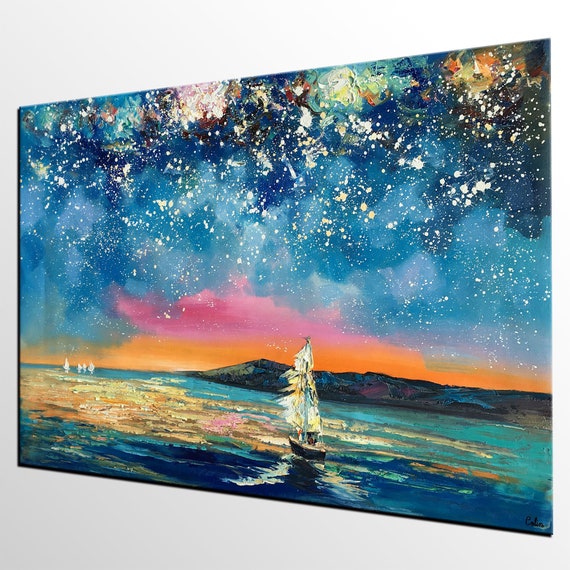This image is a highly detailed and vibrant painting of a sailboat navigating tranquil waters, prominently displaying colors reminiscent of both sunset and nighttime skies. The sail of the boat, which strikingly resembles both fire and bird feathers due to its intricate texture, features a blend of white, orange, yellow, and blue hues. The ocean beneath the boat is depicted in an abstract manner with swooshes of yellow, pink, orange, and blue tones, reflecting the colorful sky above. On the right side of the horizon, a small mountain can be seen, adding to the depth of the scene. The sky itself transitions from the fiery oranges and purples near the horizon to darker blues dotted with numerous large, bright stars, evoking the final moments of a sunset blending into the onset of night. Additional smaller boats are visible on the left side of the horizon, their white shapes barely distinguishable in the colorful expanse. The painting, set against a white wall, possibly in a museum, offers a serene yet dynamic representation of nature's beauty, with its dark cove and rocky formations further enhancing the scene.